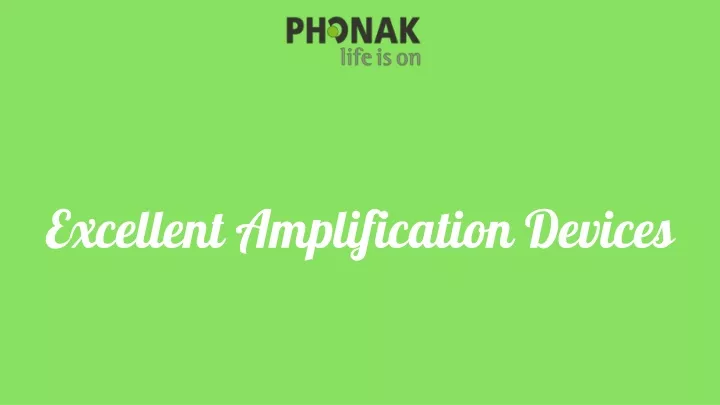The rectangular image has a bright lime green background and serves as an advertisement likely designed for the internet or a magazine. At the top center, in bold black text, it features the logo "Phonak," with a unique detail: the 'O' in Phonak contains a green dot resembling a tennis ball cut in half. Directly beneath this, in gray text, the slogan reads "Life is on." In the middle of the image, white cursive text spans from left to right, stating "Excellent Amplification Devices," with each word starting with an uppercase letter while the rest are lowercase. Despite no visual representation of the devices themselves, the clean, minimalist design strongly conveys the high-quality nature of Phonak's offerings.